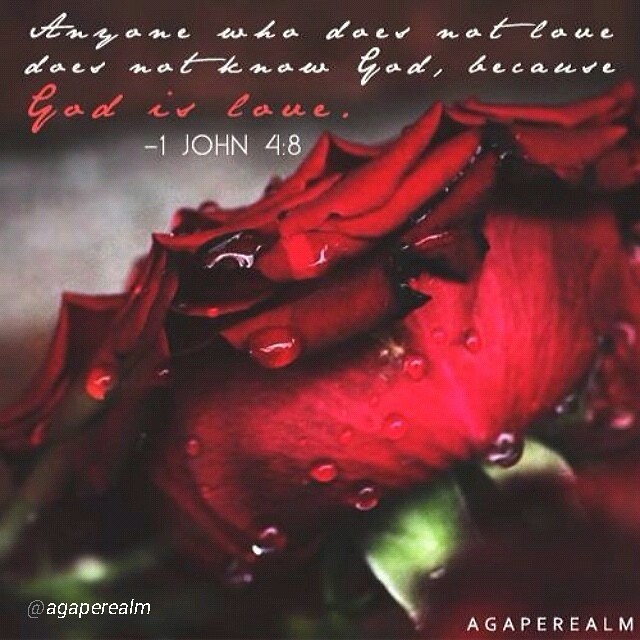The image is a square, close-up photograph of a vibrant red rose adorned with raindrops or dew, which gives it an exquisite and delicate appearance. The rose, with abundant petals at the top, dominates the center of the frame, while the green leaves and stem are visible below, adding contrast and depth. Above the rose, in a stylized cursive font, the text reads, "Anyone who does not love, does not know God, because God is love." This quote is attributed to 1 John 4:8. In the lower corners of the image, the text "Agaparelm" appears in white, with the bottom left corner including an additional "at" symbol, formatted as "@Agaparelm." The overall composition emphasizes the beauty of the flower and the poignant religious message it conveys.